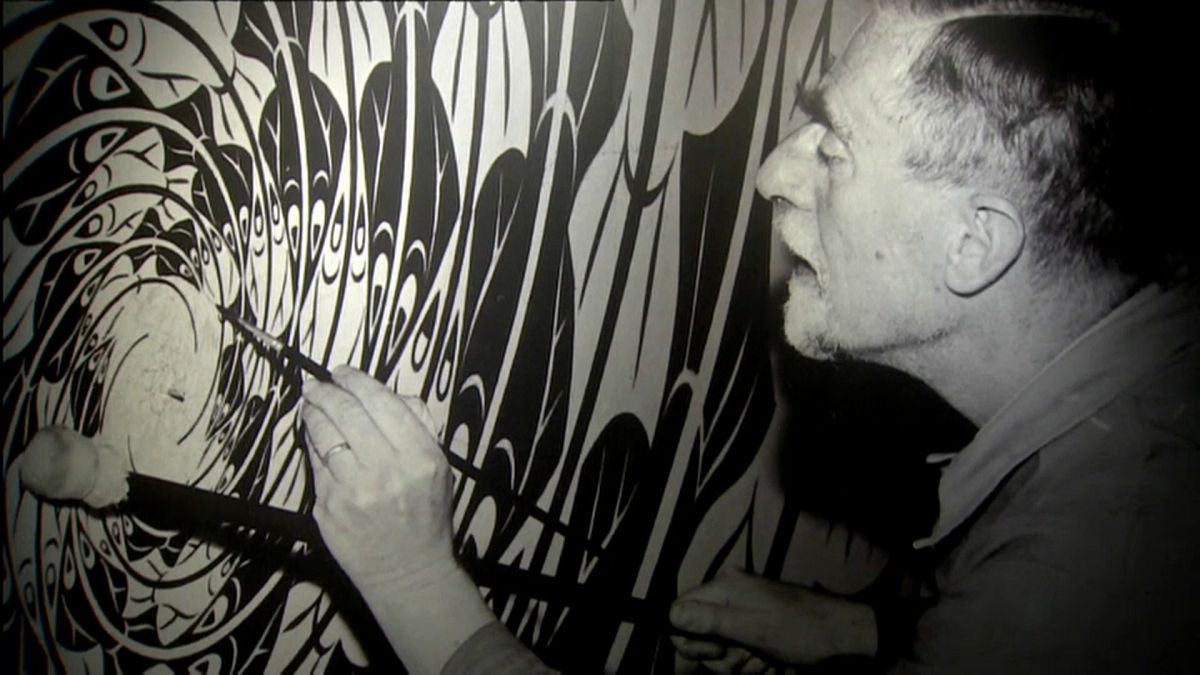This black and white photograph captures an older gentleman, possibly in his 70s, deeply engaged in the act of painting on a wall. Positioned on the right-hand side of the image, the man is portrayed in profile as he faces to the left, his focused demeanor evident. Clad in a collared shirt, he sports a slight gray beard and mustache, complemented by bushy eyebrows and short dark hair. In his extended left hand, he delicately wields a long, slim paintbrush, while his right hand grips a thicker brush-like tool, characterized by a white rag or cotton ball at its end. His wedding band is subtly visible on his left hand. The artwork he is creating features intricate, swirling patterns that resemble peacock feathers, incorporating both black and white lines that radiate outward from a small white circle at the center. The photograph beautifully captures the man's concentration as he meticulously works on this detailed and almost floral design.